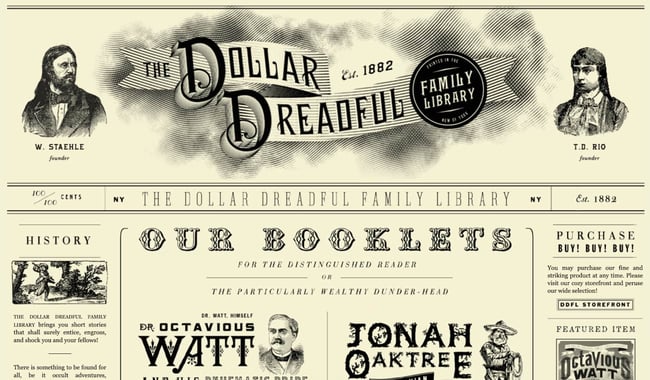The image is a detailed, old-fashioned advertisement designed to mimic a vintage newspaper or poster, featuring the "Dollar Dreadful Family Library," established in 1882. The background is cream-colored, with a rectangular shape that is approximately twice as wide as it is tall. At the top left, there's a black and white drawing of a man identified as W. Stahl, featuring long hair, a beard, a mustache, and wearing a bow tie and coat. On the right-hand side, there’s another long-haired person in a dress, possibly a woman, identified as T. D. Rio. Both figures are depicted with serious expressions and are presented in portrait form.

A ribbon-like design at the top bears the name "The Dollar Dreadful Family Library." Below this ribbon, the text announces, "Our Booklets," followed by mentions of Dr. Octavius Watt and Jonah Oaktree. Additional text includes promotional phrases like "Purchase, buy, buy, buy our booklets for the distinguished reader, or the particularly wealthy dunderhead." The entire layout uses an old-fashioned type font style and is crafted to evoke a sense of historical authenticity, despite appearing to be a modern creation inspired by vintage designs.